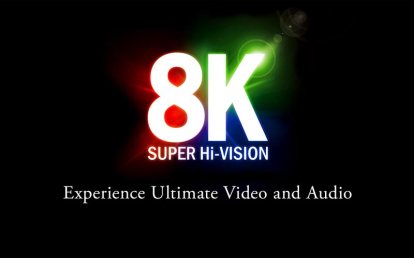This is a color image or computer-generated logo set against a solid black background. Dominating the center, the large white characters "8K" are prominently displayed. A burst of colors emerges from behind these characters, with red radiating from the left, green from the upper right, and blue from the lower right, creating a dynamic effect. Directly beneath "8K," in a smaller white font, are the words "Super High Vision," followed by "Experience Ultimate Video and Audio" in the same white font below that. An interesting detail is the subtle orb-like glow at the tip of the K, where the green light originates. The overall minimalistic design, with its stark contrast between the vibrant colors and the black background, emphasizes the logo's message of advanced video and audio quality, likely intended for use on a web page or in a manual.